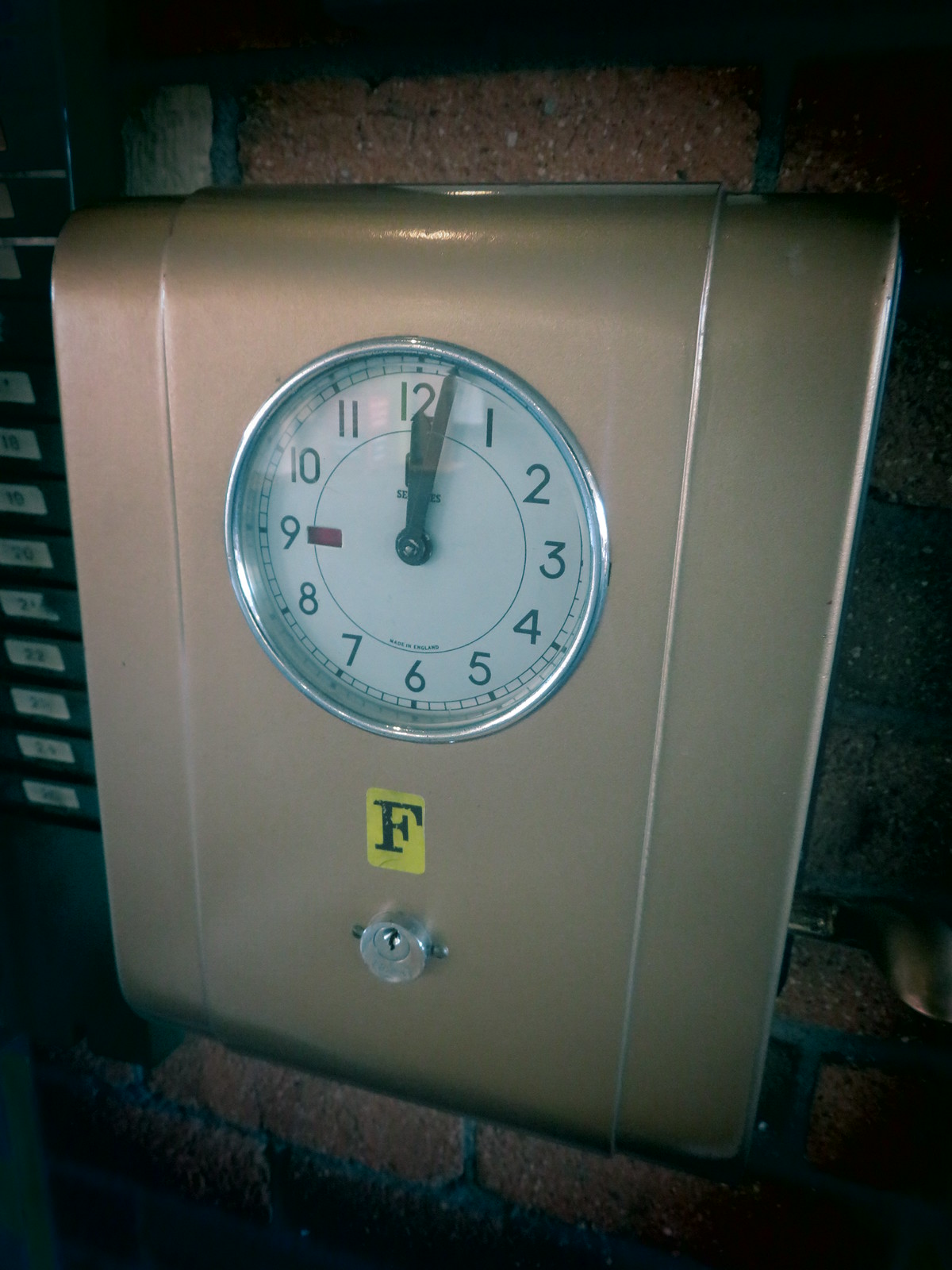In this real-life photograph, the centerpiece is a rectangular object resembling a suitcase, prominently featuring a circular clock. The clock is encased in a chrome ring, with a see-through cover that reflects light, indicating some glare. The clock face is set against a white background and displays numbers from 1 to 12, accompanied by small dashes marking each minute along the outer ring. The clock hands are black and currently show the time as 12:02. Text is faintly visible inside the clock, with an unreadable logo positioned behind the clock hands and partly decipherable text at the bottom that reads "Made in...," with the remaining portion indistinct.

Below the clock, on the rectangular object, is a distinctive yellow square featuring a black letter "F," and beneath this square, there is a small keyhole lock. The object is situated on a brick surface, with more bricks visible in the background. To the left, a partially visible object with white rectangles is cut off by the edge of the image, making it unidentifiable. The photograph is predominantly dark around the edges, suggesting the scene is in a dimly lit area, with the main light source focused on the rectangular object with the clock.